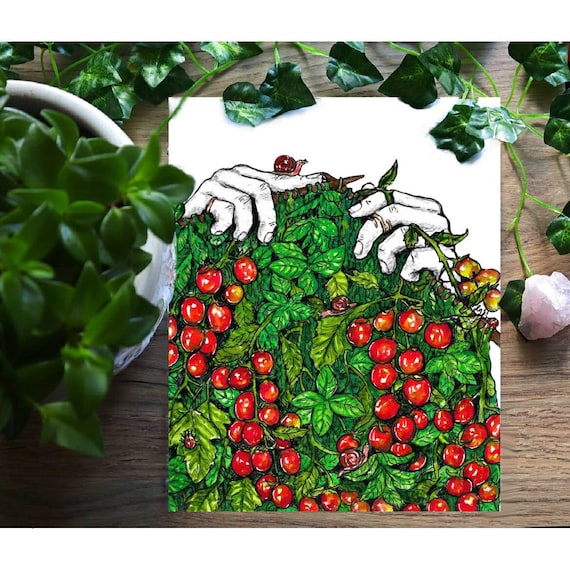The image shows a highly detailed watercolor illustration on a white sheet of paper, which is laid flat on a wooden table. The artwork depicts two hands with white fingers, one of which has a small red snail on it, crocheting grape vines and clusters of glossy red cherry tomatoes. Another red snail and a little ladybug are also visible crawling on the vibrant green leaves. The drawing is surrounded by artificial ivy with small pink flowers at the top. To the left of the artwork, there is a potted plant with green foliage, and to the right, a piece of pink quartz sits near the edge of the image. The entire composition blends natural elements with the delicate intricacies of the illustration, creating a harmonious and rich visual experience.